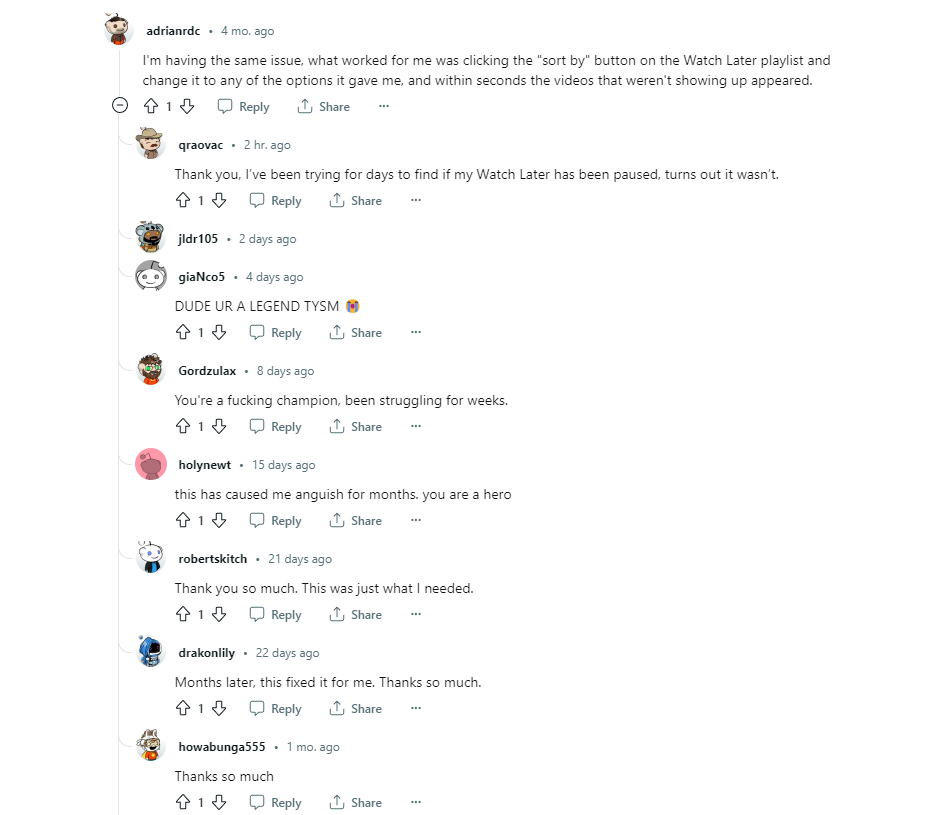"An image features a lively conversation thread filled with gratitude and relief from numerous users. It all started when one person shared a solution to an issue with the 'Watch Later' playlist. Their instructions to click the 'Sort by' button and change it to any available option led to videos appearing that had previously been missing. The thread quickly filled with heartfelt thanks, such as: 'Thank you, I've been trying for days to fix this,' 'You’re a legend, thank you so much,' and 'You are a hero. You've ended my weeks of struggle and anguish.' Several users also referred to the solution provider as a 'champion' and 'hero,' expressing immense gratitude for the effective fix. Notably, each user in the conversation has a profile picture represented by a unique cartoon face, creating a vibrant and cohesive visual theme throughout the thread."